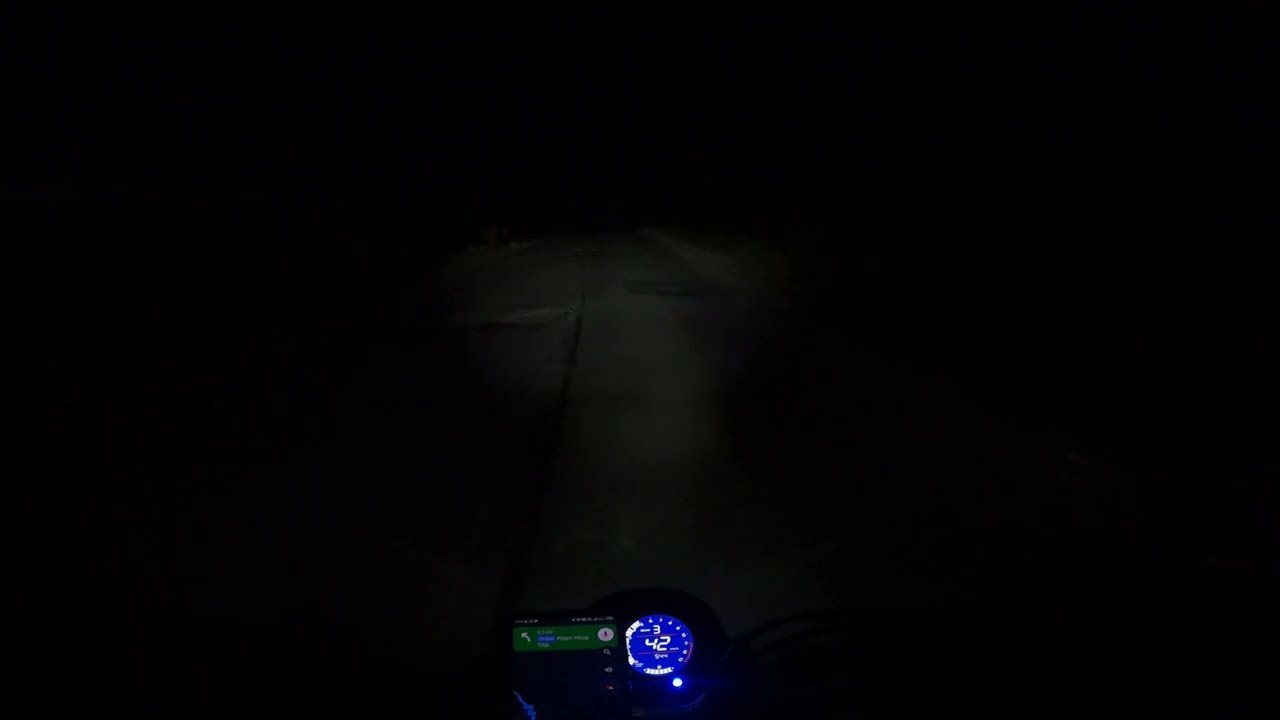This image captures a nighttime scene of a motorcycle traveling on a dimly lit road. The center is dominated by a bright blue speedometer displaying the number 42 in white. To the left of the speedometer, there is a green GPS display indicating a left turn, with small icons and possibly an audio button visible. The motorcycle's handlebars are partially seen, adding to the realism of the scene. Illuminated by an LED light, the road ahead is faintly visible, while the surroundings fade into darkness. The general aesthetic suggests a sense of solitude and focus, as the rider navigates through the night, framed by a predominantly black background.